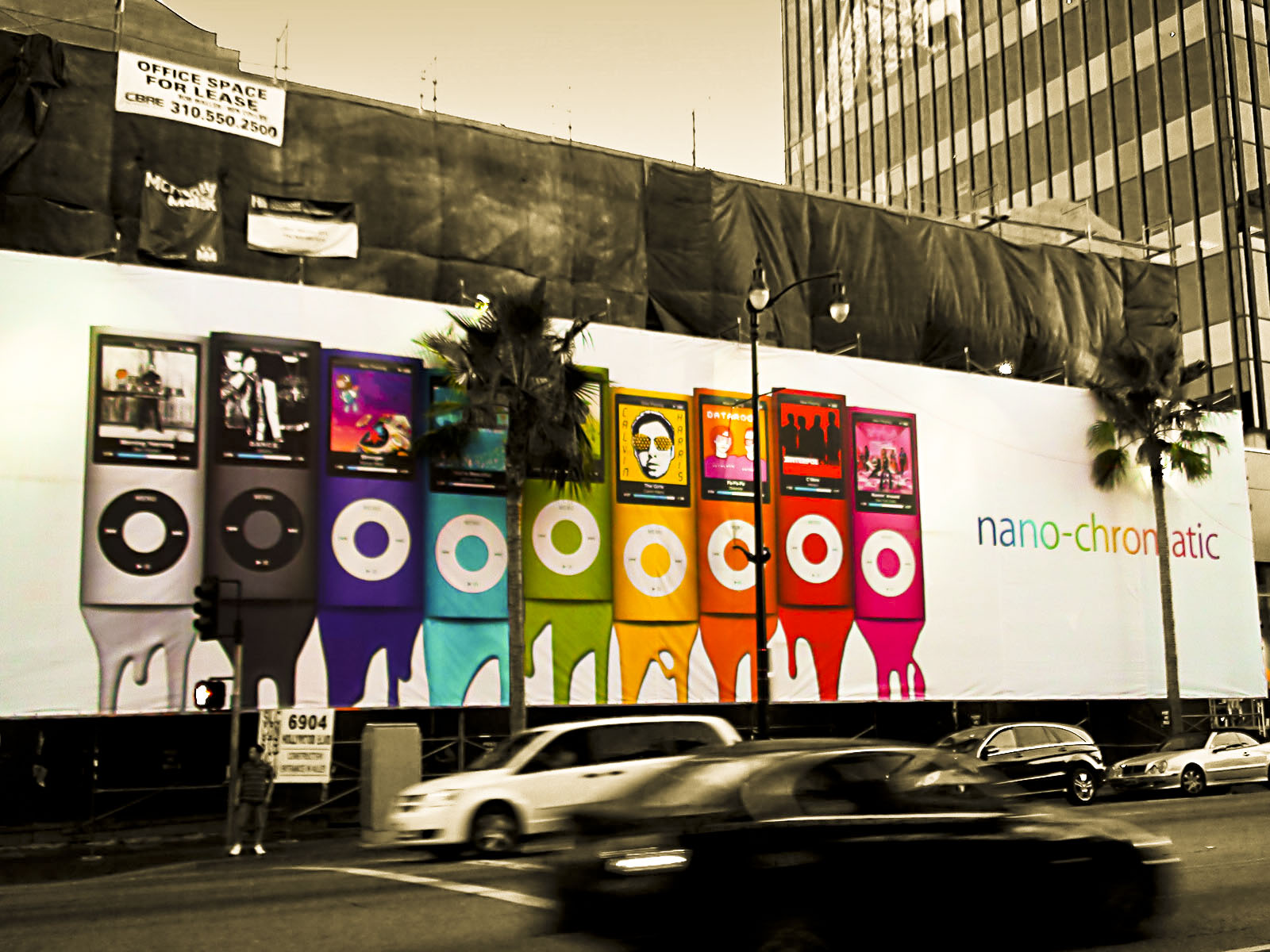In this striking image, we observe a large advertisement prominently displayed on the side of a building, functioning as a colorful billboard in an otherwise black and white scene. The entire environment, including the buildings, cars, street, and even the trees in front of the billboard, is rendered in monochromatic tones, creating a stark dichromatic contrast. The focal point of the advertisement is an old-school iPod, reminiscent of models from 2006 or 2007, featuring buttons and a small colored screen. The iPods are displayed in a variety of vibrant colors, standing out vividly against the grayscale backdrop. Adding to the visual appeal, there is text on the billboard that reads "nanochromatic," adorned in a vibrant, rainbow font, emphasizing the burst of color in an otherwise subdued setting.